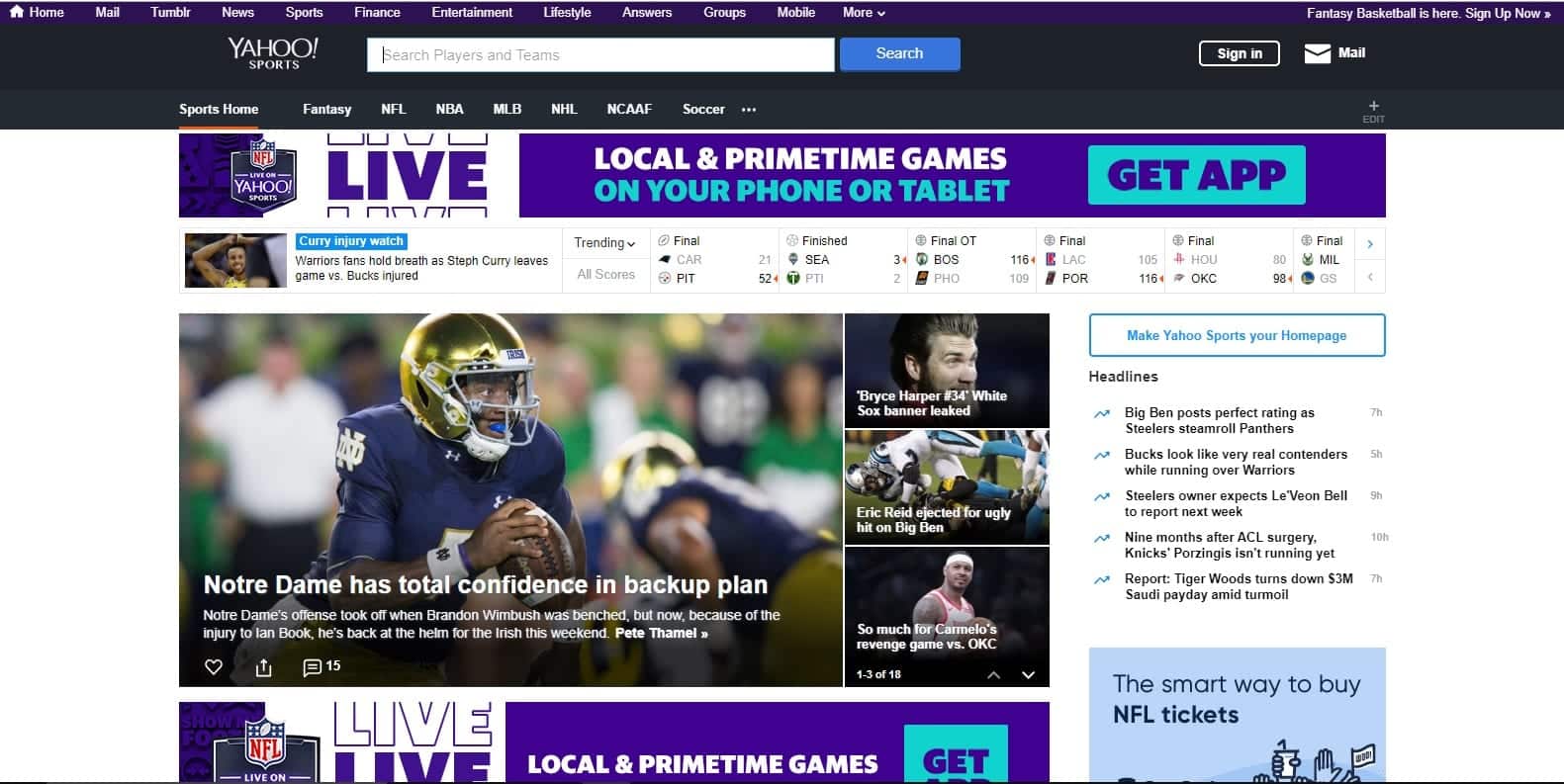The image features a Yahoo Sports webpage. At the top, a black bar extends wider than the actual website, displaying the Yahoo Sports logo along with various functional elements. On the left side, there's a search bar, allowing users to type in queries. To the right of this bar, a blue button prominently labelled "Search" allows users to initiate the search. 

Next to these elements, various user options are displayed, including "Sign In" and "Mail." Below this top bar, a navigation menu lists different sports categories such as NHL, NFL, NBA, etc. A colorful banner in shades of purple, blue, and white announces "Live local and primetime games on your phone or tablet" with a call-to-action button labeled "Get App" in purple within a blue rectangle.

Beneath this banner, there is an image of a football player in action, accompanied by some statistics. Directly below, another image depicts a football player from Notre Dame wearing a gold helmet and blue uniform. The caption reads, "Notre Dame has total confidence in backup plan," followed by a brief summary about the player.

Adjacent to this, three smaller images of different athletes are displayed, each with a short description or caption. At the bottom of the image, the phrase "Live local and prime games" is reiterated. Another "Get App" call-to-action button appears, and next to it, a blue box with the message "A smart way to buy NFL tickets" is displayed.

This detailed structure effectively showcases how Yahoo Sports enables users to stay connected with live games, player stats, and NFL ticket purchases.